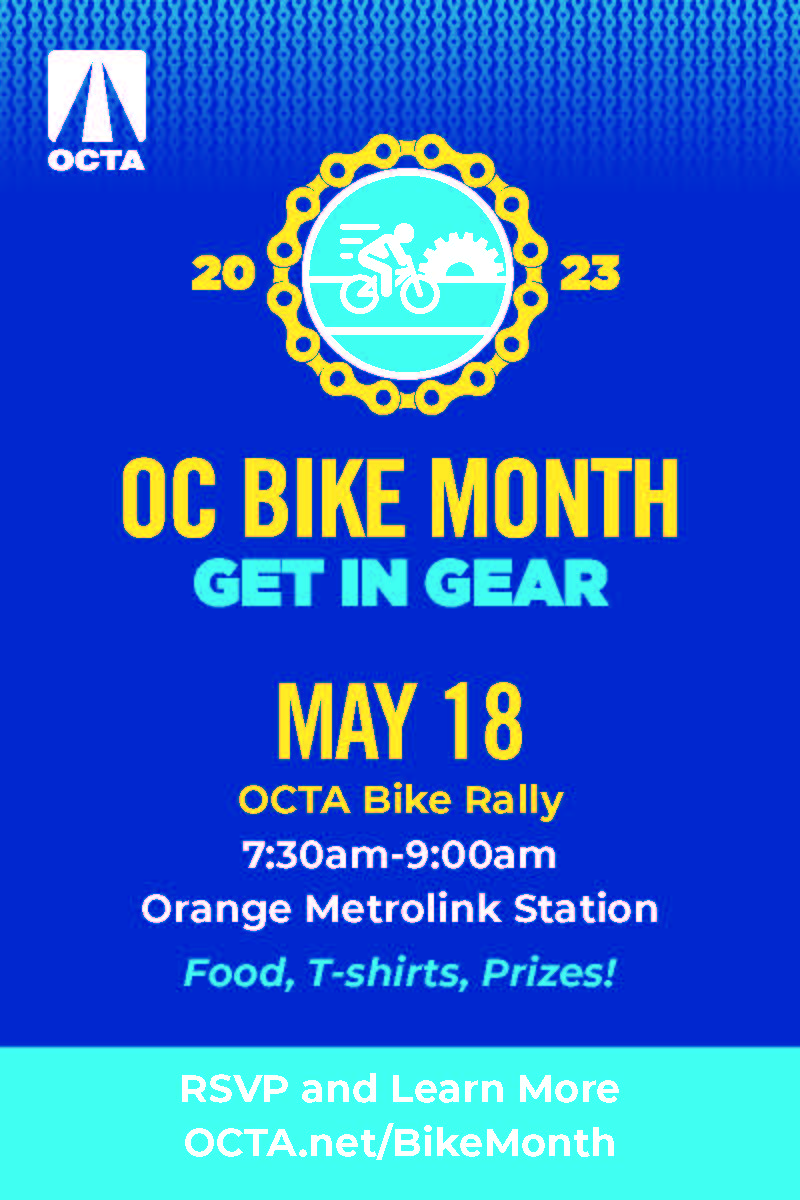The image is a detailed promotional flyer for the 2023 OC Bike Month "Get In Gear" event. The background is predominantly dark blue, accented with a lighter blue chain pattern at the top and an aqua-colored band at the bottom. Central to the design is a prominent logo at the top, featuring a cyclist speeding down a path with a gear-shaped sun in the background, encircled by a gold bike chain. The numbers "20" and "23" flank this logo. In the top left corner, there's another logo depicting railway tracks receding into the distance, with "O-C-T-A" inscribed below it in white. The text on the flyer is primarily in gold, aqua, and white, detailing the event specifics: "OC Bike Month," "Get In Gear," "May 18th OCTA Bike Rally," and the timing "7:30 a.m. to 9 a.m." at the "Orange Metrolink Station." Additional information includes "Food, T-Shirts, Prizes," and a call to action to "RSVP and Learn More at Octa.net/BikeMonth," written in aqua with white text.